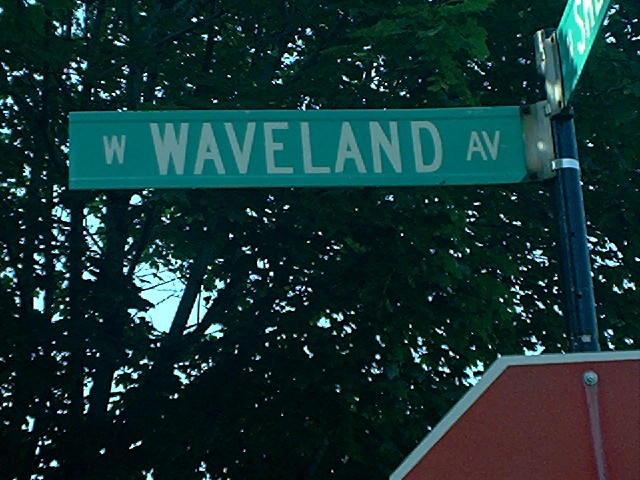A vibrant daytime photograph captures a tranquil street scene, dominated by a green street sign that reads "Waveland AV" in bold white letters. The street sign is prominently positioned in the top right corner and is brightly lit by daylight, providing a striking contrast to the blue pole it is mounted on. Below the street sign, and in the bottom right corner, portions of a stop sign are visible, revealing only the red color and white edging. The background consists of a dense canopy of trees, casting deep shadows that render the foliage dark, while glimpses of a pale blue and light gray sky peek through the gaps in the leaves, adding a subtle, serene backdrop to the image.